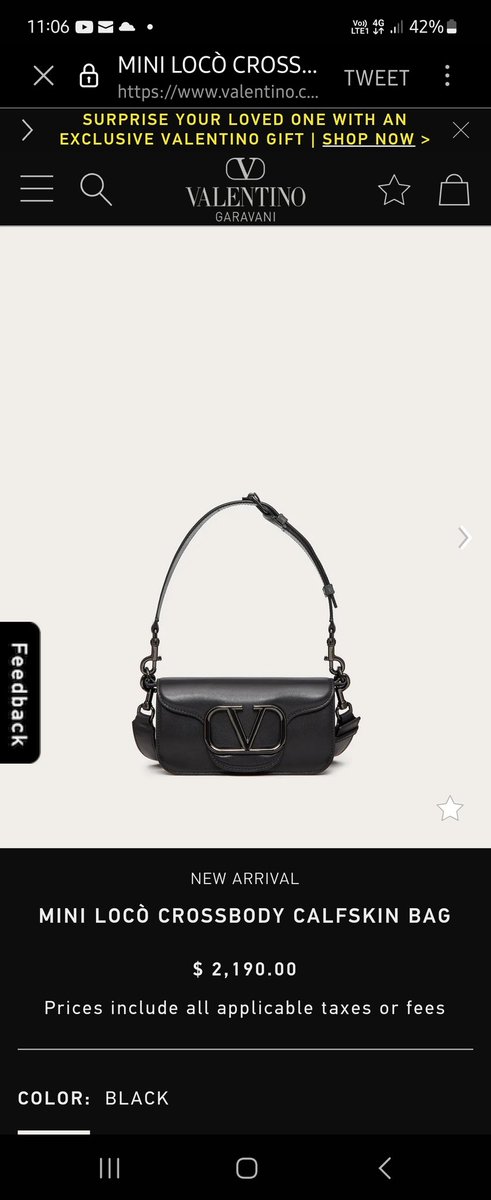This image is a portrait-mode screenshot depicting a mobile shopping interface for Valentino. At the top left corner, the time is displayed as 11:06, accompanied by icons for a video, an envelope, and a cloud. The right-hand side shows a battery percentage at 42%. Below this row, there is a close (X) button and a secured icon followed by the text "Mini Loco Cross." The URL bar reads "Valentino," while to its right, there is a tweet button and a three-dot menu. 

Beneath the URL bar, a gray horizontal line spans the screen, followed by a right arrow on the left. In bold yellow text against a black background, the message "Surprise your loved one with an exclusive Valentino gift. Shop now" is highlighted, with the "Shop now" text underlined. An X icon is located to the right of this message.

Below, a navigation bar features three horizontal lines (menu), a search bar, and the Valentino Garavani logo. To the right are icons for favoriting (star) and an empty shopping cart. 

The background then transitions to a cream color, displaying an image of a Valentino bag. A vertical "Feedback" button is on the left side. 

At the bottom, the background changes back to black, showcasing the item details: "New Arrival Mini Loco Crossbody Calf Skin Bag," priced at $2,190. It includes a note that prices encompass all applicable tees, taxes, or fees, and specifies the color as black.